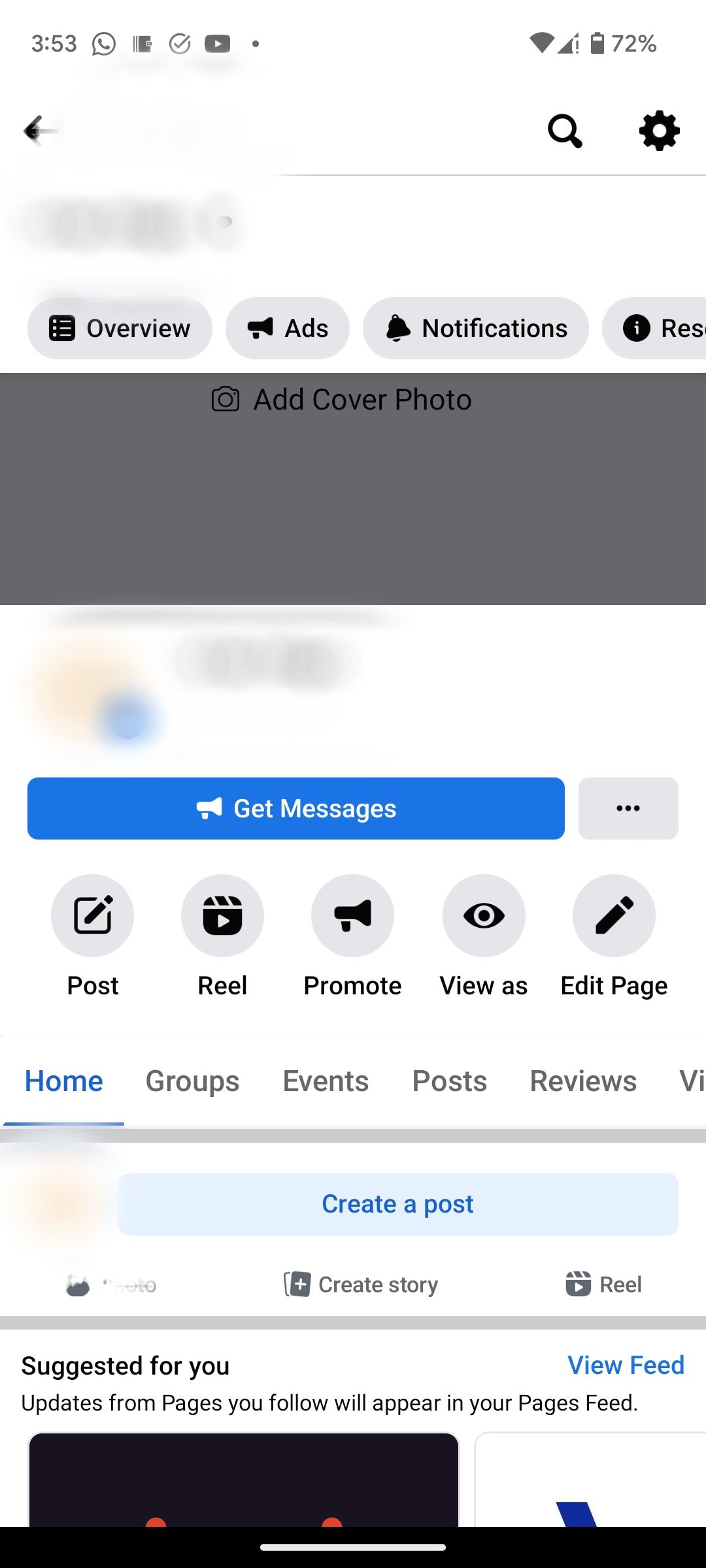This image is a screenshot from a mobile device displaying a Facebook page with a white background. At the top of the page, there's a section that is blurred out. On the right side, visible icons include a search button and a settings gear. Below this, there are four gray bubbles labeled from left to right: "Overview," "Ads," "Notifications," and "Reset." 

Continuing down, there is a section for adding an ad photo cover, followed by options labeled: "Get Messages," "Post," "Reel," "Promote," "View As," and "Edit Page." Below this, there are tabs for "Home," "Groups," "Events," "Post," "Reviews," and a partially visible "Videos" tab. Further down, there's a "Create a post" section with another blurred area to its left. At the bottom of the screenshot, there is a section titled "Suggested for you" followed by a "View Feed" button.